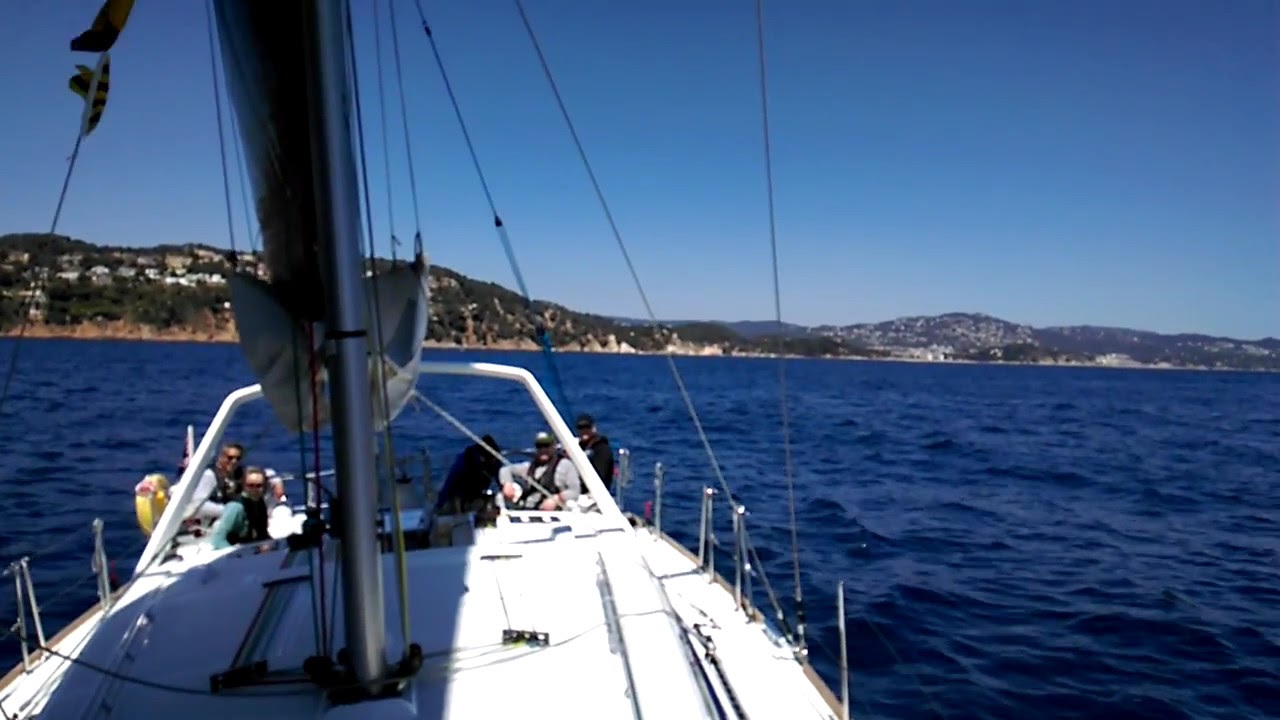The image captures a large white sailboat with its sails rolled down, occupying much of the bottom left portion of the frame. The boat, mostly in shadow cast by its mast, has five people sitting in the piloting area. Among them, a man in an aqua shirt and life vest is identifiable, while another person in white shorts is bending over. Metal poles with wires act as railings on either side of the boat. The boat is sailing on a dark blue, clean, and slightly wavy body of water. In the distance lies a vast expanse of green and brown hills dotted with numerous gray and white rectangular buildings, suggesting a sizeable waterfront city. To the right, several mountains rise under a cloudless sky transitioning from light to dark blue. The weather appears pleasant, with some individuals in short sleeves, indicating a warm, enjoyable day out on the water.